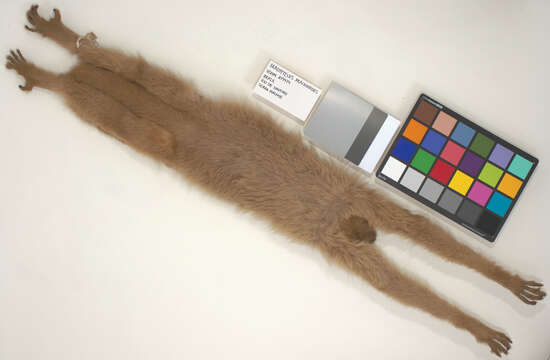The photograph features the skin of a small, brown-furred animal, possibly a monkey, laid out on a white table. The animal’s skin is stretched diagonally from the top left to the bottom right, with its front legs extending towards the top left corner and its back legs towards the bottom right. Notably, the head is missing. Positioned above the animal skin, there is a colorful palette reminiscent of an eye shadow collection or an art palette, containing squares in an array of hues including browns, pinks, blues, greens, yellows, and blacks. To the left of this palette is a plastic object in shades of gray, black, and white, whose purpose is unclear, and a white piece of paper with black text that is illegible due to photo compression and low resolution. The overall scene evokes a sense of oddity, as if comparing the fur’s color to the palette.